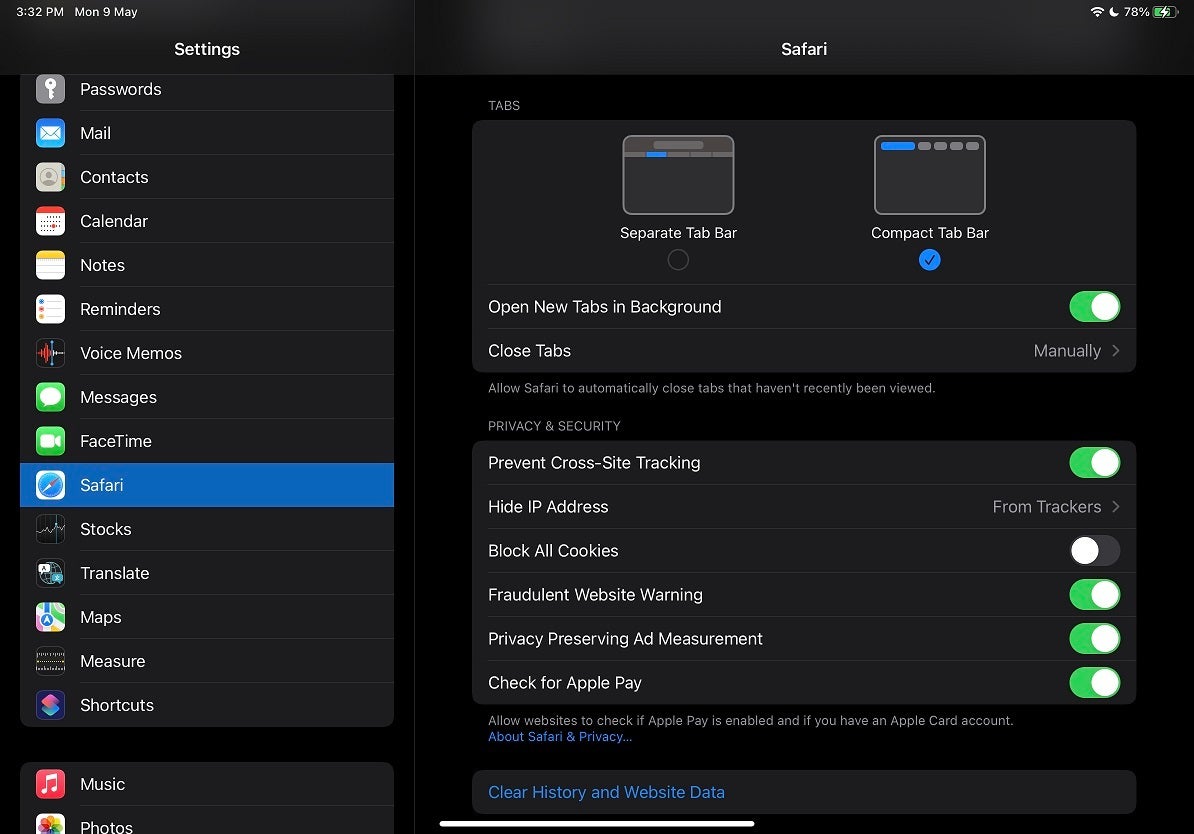This is a detailed screenshot of an iPad in landscape orientation, displaying the settings app in dark mode under the Safari tab. The top left corner of the screen shows the current date and time: 3:32 PM, Monday, 9th of May. In the top right corner, the status bar indicates full Wi-Fi signal, the Do Not Disturb icon, and a battery level of 78% with the device currently charging.

In the Safari settings, the Tabs section highlights that the Compact Tab Bar is enabled instead of the Separate Tab Bar. Also, the "Open new tabs in background" option is turned on, and "Close tabs" is set to "Manually." A description below clarifies that this setting allows Safari to automatically close tabs that haven't been recently viewed.

In the Privacy & Security section, several settings are adjusted for enhanced security and privacy:
- "Prevent Cross-Site Tracking" is turned on.
- "Hide IP Address" is set to "From Trackers."
- "Block All Cookies" is turned off.
- "Fraudulent Website Warning" is turned on.
- "Privacy-Preserving Ad Measurement" is turned on.
- "Check for Apple Pay" is turned on, which allows websites to verify if Apple Pay is enabled and if the user has an Apple Card account.

At the bottom of the Privacy & Security section, there is a link titled "About Safari & Privacy," and the final button, "Clear History and Website Data," is prominently displayed in blue text, offering a quick way to clear browsing data.